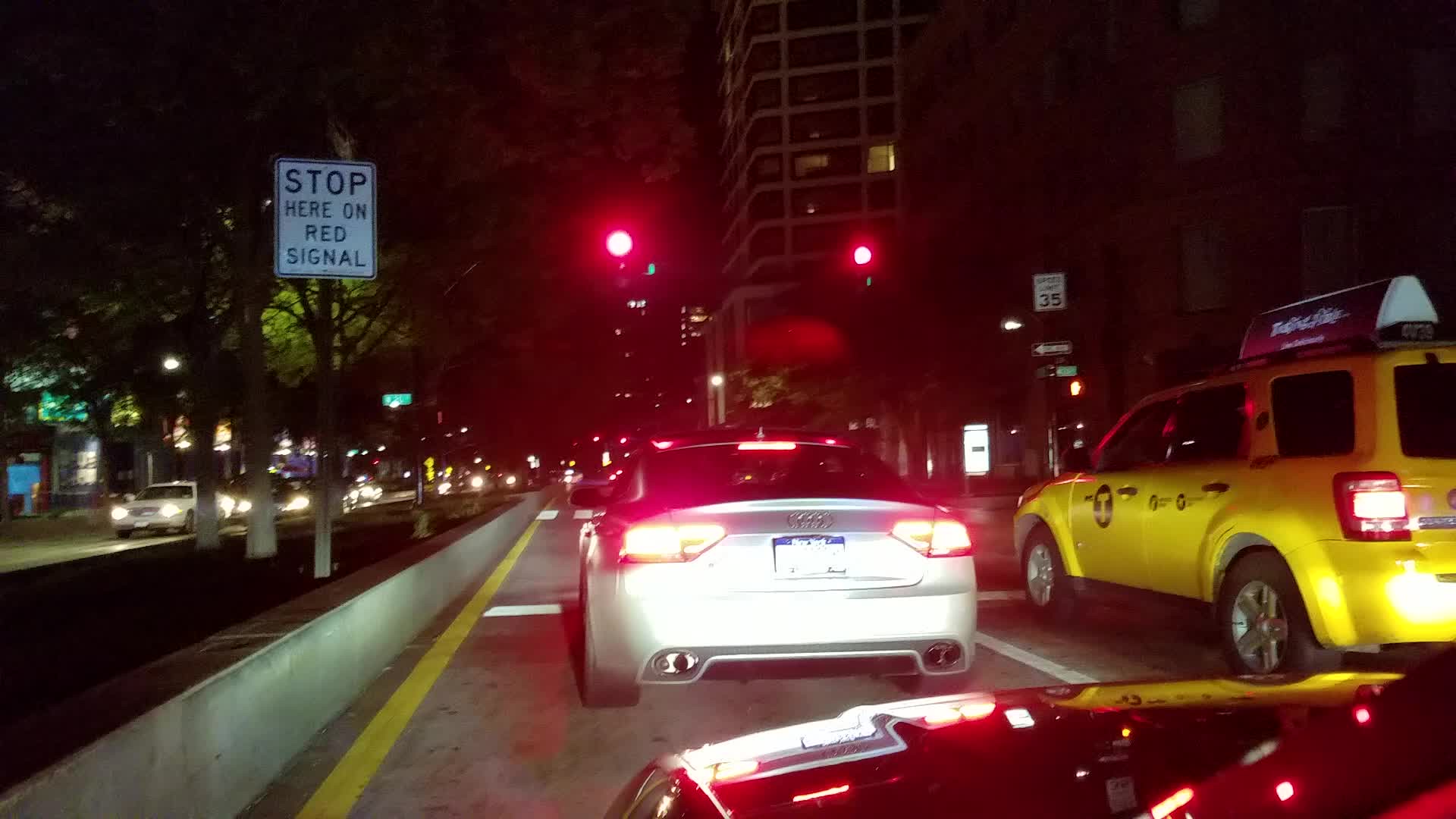This photograph captures an urban street scene at night, taken from inside a car that’s stopped at a red light in a downtown area. The vehicle, whose color could be red or black, is the second in line behind a silver Audi, which appears to have a dealer tag. To the right of the Audi is a yellow taxi SUV, possibly a Chevy, featuring a logo on its driver's door and an advertisement on its roof. A traffic sign in the left foreground reads, "Stop here on red signal" and stands out against the backdrop of dimly lit trees located in a median divide. Across the median, several cars with headlights on are waiting in the opposite direction. The median itself is about six to eight feet wide, reinforced with low concrete walls to prevent cars from crossing into oncoming traffic. In the distance, tall office or residential buildings loom, epitomizing the urban setting. Reflections from the streetlights create a vivid interplay of light on the vehicles and surrounding structures.